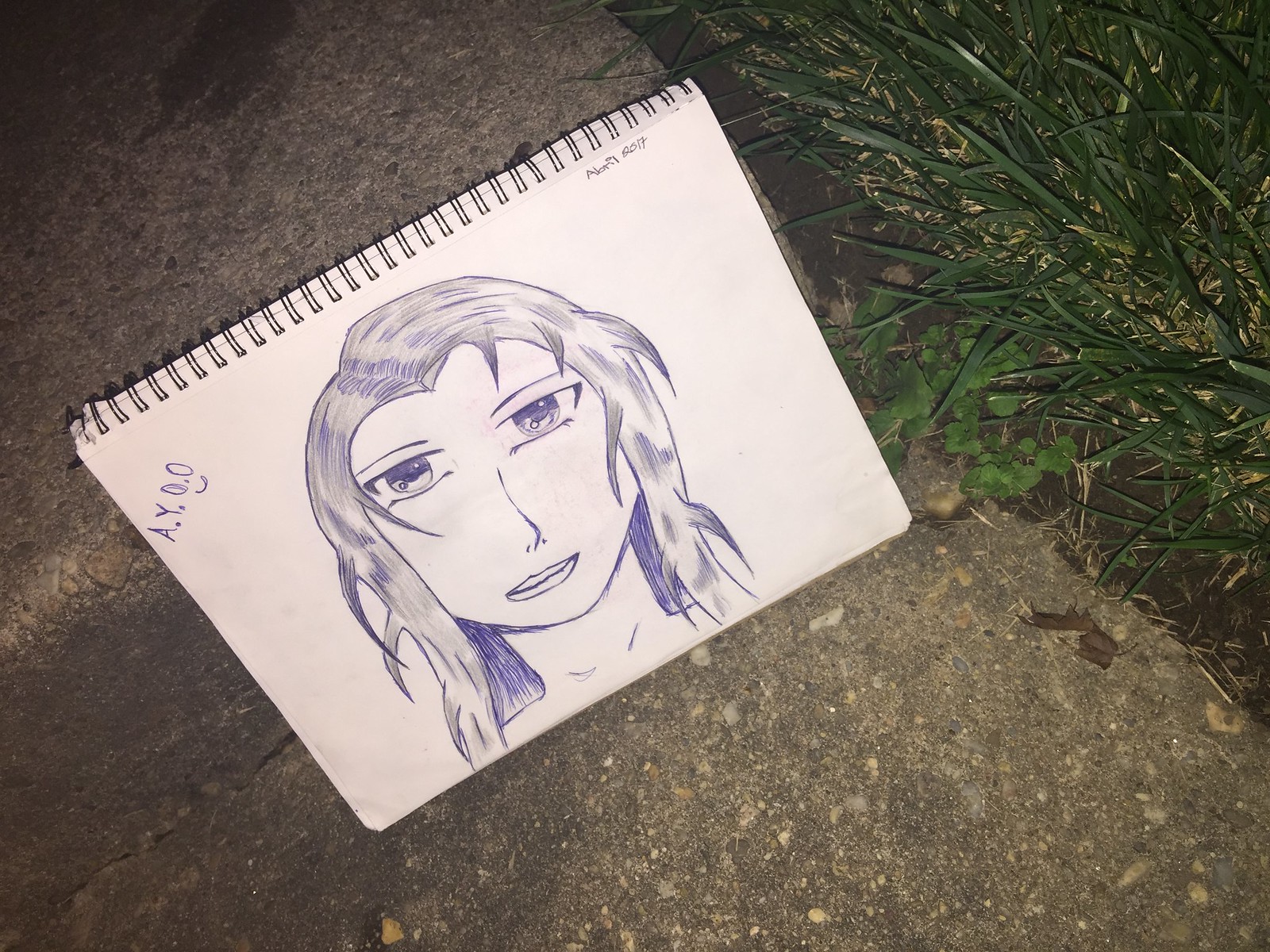A photograph captures an illustration in someone's sketchbook, placed outdoors in the evening under dim light conditions. The scene is predominantly dark, cast in deep shadows, with the only apparent light sources being the camera's flash and possibly another artificial light to the left, barely illuminating parts of the ground. The sketchbook is situated on a sidewalk or pavement, with a patch of grass visible on the right side of the path. The sketchbook itself is rectangular with the longer sides positioned at the top and bottom, bound by black spiral wires. The paper is strikingly white and is folded to stand upright on the pavement. The featured illustration appears to be meticulously drawn in ballpoint ink.